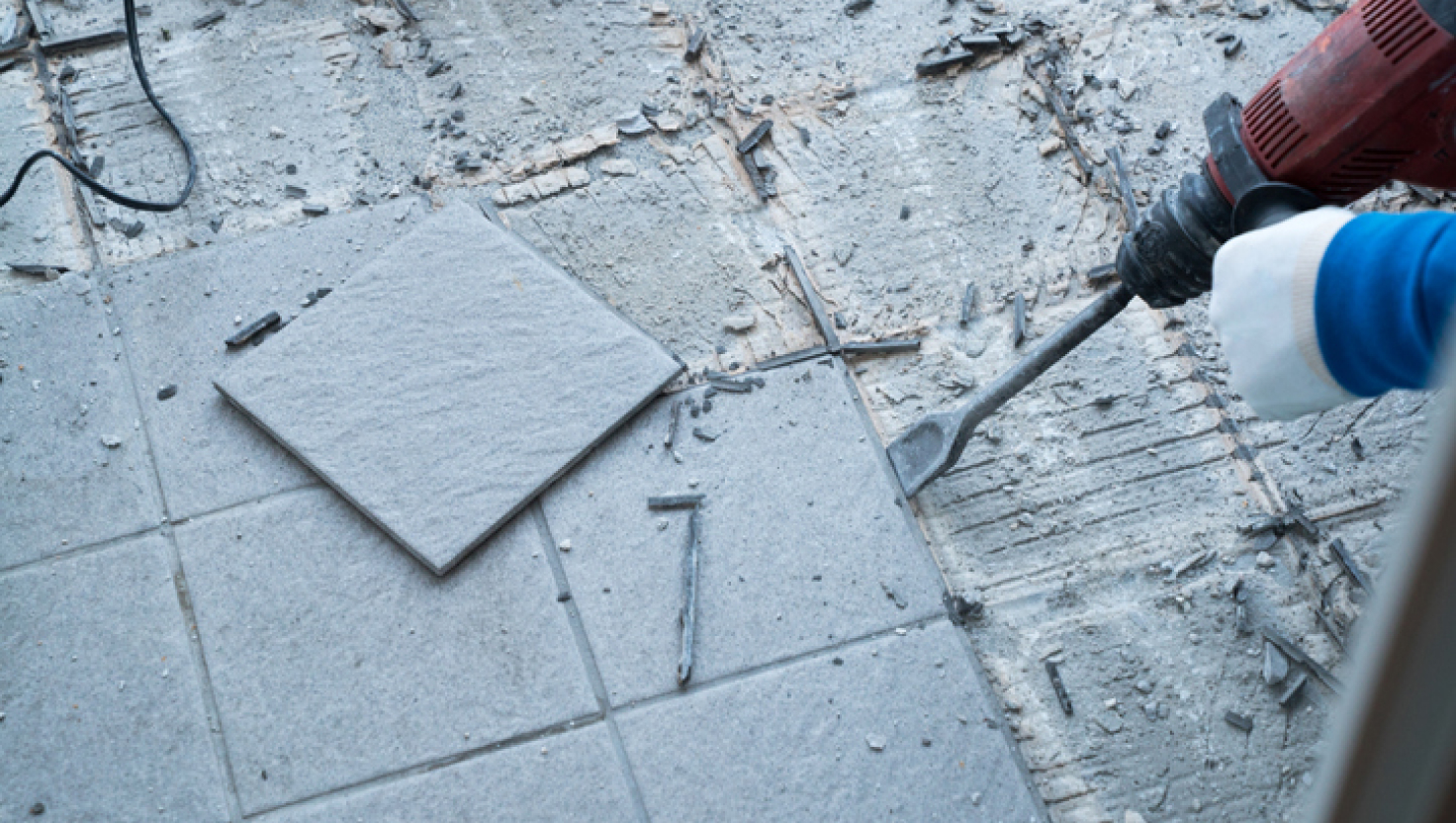The photograph depicts a detailed scene of a man jackhammering tiles off a floor, revealing the underlying concrete. The floor features a mix of intact gray slate tiles and an exposed, rough concrete area where tiles have been removed, showcasing a square pattern from the adhesive residue. The man, only partially visible, is dressed in a long-sleeved blue shirt and white gloves, holding a well-worn red jackhammer with black trim and a dull gray metal chisel attachment. A black power cord, not fully visible, extends from the top left of the image. The jackhammer's faded red body and weathered appearance indicate extensive use, while the gray chisel end, resembling a spatula, is actively engaged in lifting a tile. The removal process appears to be more than halfway complete, with most of the remaining tiles situated at the bottom and left sides of the image.